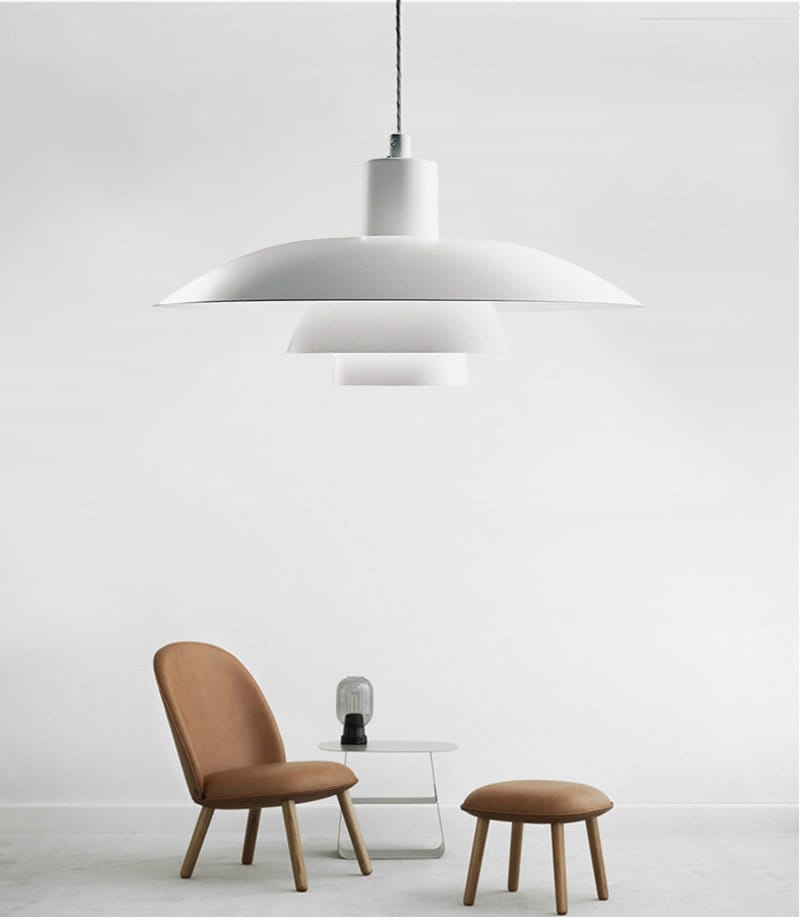The image captures a very modern and minimalist living area dominated by a strikingly large white hanging lamp, which creates a sense of scale and takes up the upper third of the photo. The lamp comprises three descending sections, becoming narrower towards the bottom, almost resembling an inverted triangle or tiered structure. The backdrop is stark and clean with an entirely white wall, complemented by a slightly darker white floor, maintaining the minimalist aesthetic.

Central to the lower portion of the image is a simple white table with a distinctive curved design that merges into the floor, devoid of traditional legs. Atop this table is an old-fashioned oil lantern featuring a black base and a clear glass top. Positioned on the left is a light brown chair with wooden legs, offering a cozy yet modern seating option. In line with the chair in the middle right is a matching brown footstool, maintaining the minimalist theme.

Adding to the simplicity of the arrangement, there is a minimalist, open bookshelf or shelf near the chair, enhancing the room's functionality while keeping the design uncluttered. The overall composition emphasizes a serene, almost empty space where each piece of furniture serves both form and function, conveying a sense of tranquility and refined modernity.